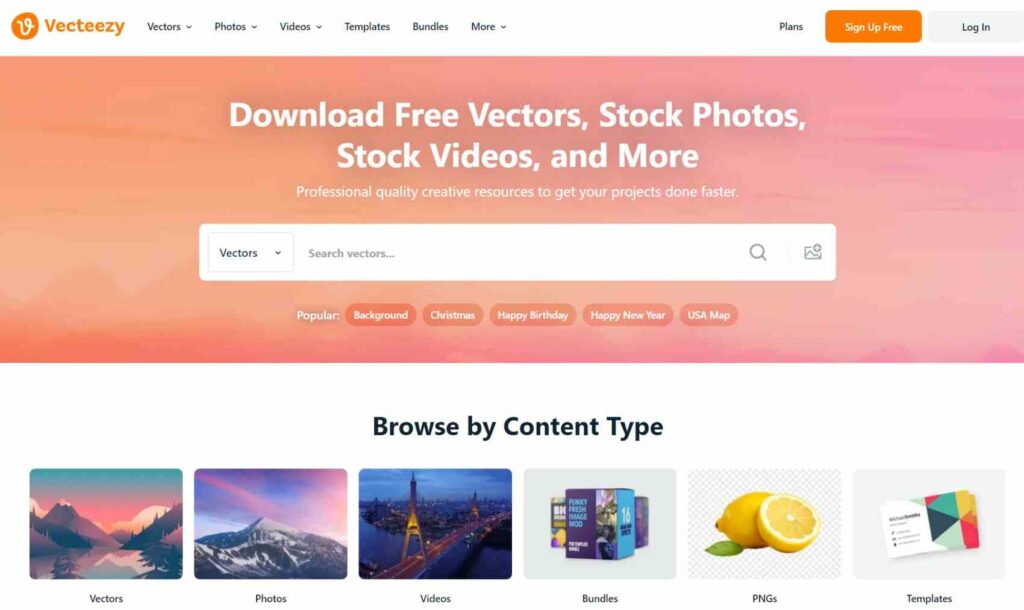The image features a clean, solid white background. In the upper left corner, there is orange text that reads "Vecteezy," accompanied by an orange logo to its left consisting of a 'V' inside an orange circle. To the right of this text, in black, are the words "Vectors, Photos, Videos, Templates, Bundles, and More." 

In the upper right corner of the image, there are prompts for user engagement: "Sign Up for Free" and "Log In." Positioned below this is a vibrant banner blending orange and pink hues. On this banner, white text proclaims, "Download Free Vectors, Stock Photos, Stock Videos, and More. Professional Quality, Creative Resources to Get Your Projects Done Faster."

Directly beneath this banner is a white search bar with a dropdown menu labeled "Vectors" on the left, and the text "Search Vectors" within the bar. Below the search bar are popular search keywords listed as "Popular, Background, Christmas, Happy Birthday, Happy New Year," and "USA Map."